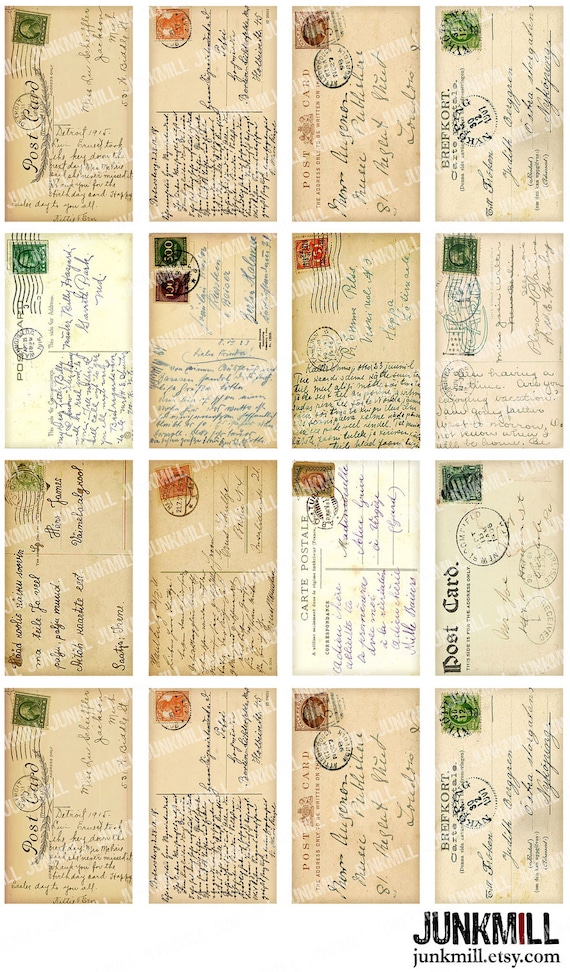This photograph showcases a meticulously arranged collection of 16 vintage postcards, each laden with history and character. The postcards are displayed in a 4x4 grid, with their longer sides vertically aligned, making the array taller than it is wide. They rest against a clean white background. Each postcard is weathered, showing various stages of aging, from yellowed hues to darker browns. Handwritten cursive text adorns the postcards, many of them bearing the word "postcard" at the top, while some display "carte postale," hinting at their French origin.

Every postcard features at least one postage stamp in the upper right corner, with a range of colors including green, brown, and orange. Notably, one postcard in the second row bears two stamps, distinguishing it from the rest. The stamps and postmarks imply these postcards were once mailed from different locations.

In the bottom-right corner of the photograph, a logo reads "Junk Mill" with a distinctive red "I" amidst black letters. Directly below this, the website "junkmill.etsy.com" is printed in smaller black letters. The entire arrangement evokes a sense of nostalgia and curiosity, offering a visual journey through past correspondences.